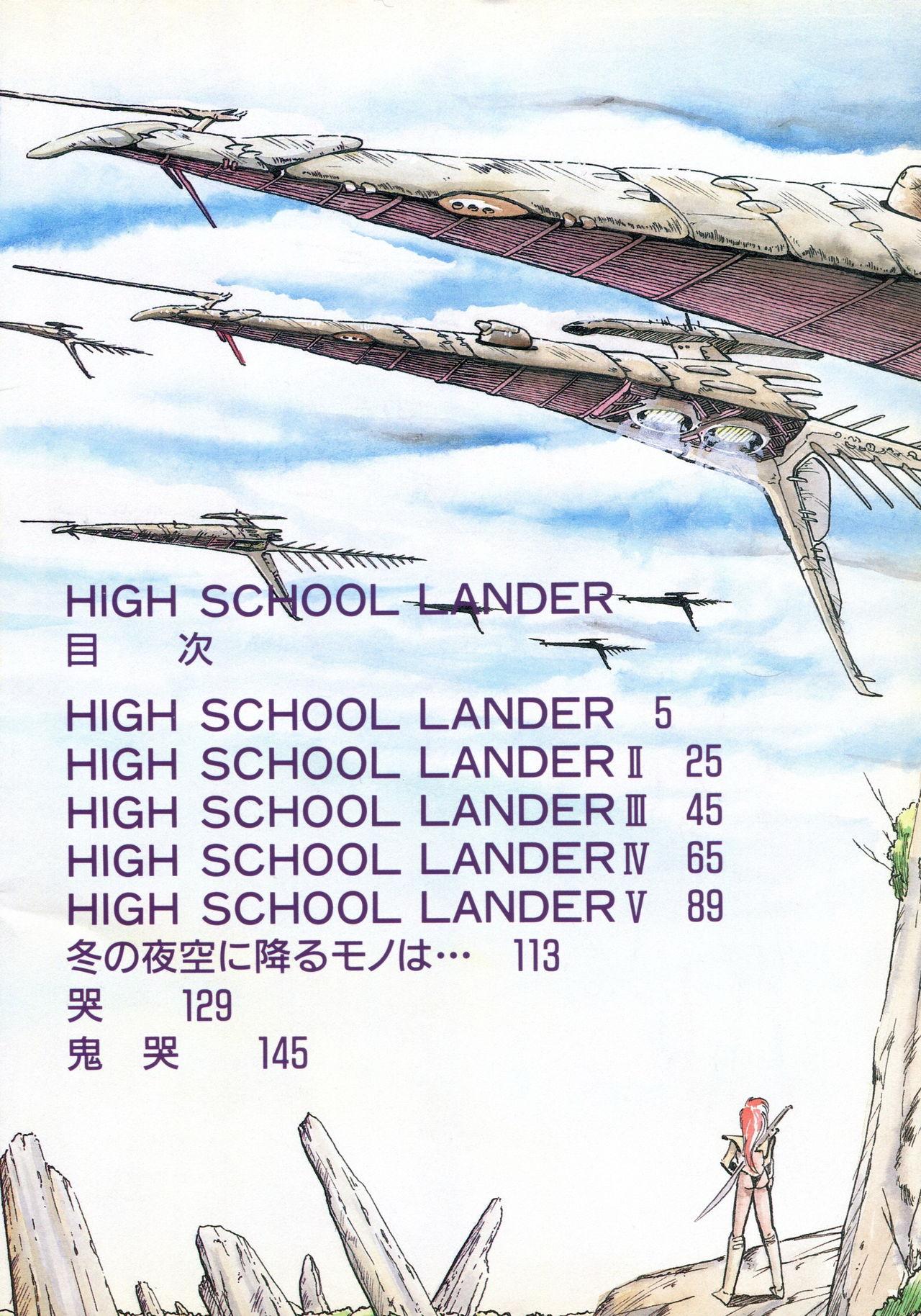The horizontally aligned, borderless anime poster features a sketched, animated scene set against a primarily white background with hints of blue sky and fluffy white clouds near the top. Dominating the upper part of the image are five brown fighter jets, their tips facing left, soaring through the sky at different altitudes, with the three distant jets appearing smaller. In the foreground, a small female figure with long reddish hair stands on a rocky cliff on the lower right, brandishing a sword on her back. She is dressed in tall boots and what appears to be a thong, with her back turned towards the viewer. The rocky terrain around her is interspersed with dead tree stumps and a lone dead tree with a bit of green foliage beside her.

Centered in the image are several lines of brown text, starting with "High School Lander" and followed by various Roman numerals and numbers: 
- "High School Lander V," "25"
- "High School Lander II," "45"
- "High School Lander III," "65"
- "High School Lander IV," "89"
- "High School Lander V," "113"

Below these inscriptions are three rows of symbols, possibly Chinese or Oriental characters, each accompanied by corresponding numbers: 
- "113"
- "129"
- "145"

This intricate scene combines elements of a post-apocalyptic landscape with futuristic aerial dynamics, all united under the title "High School Lander."